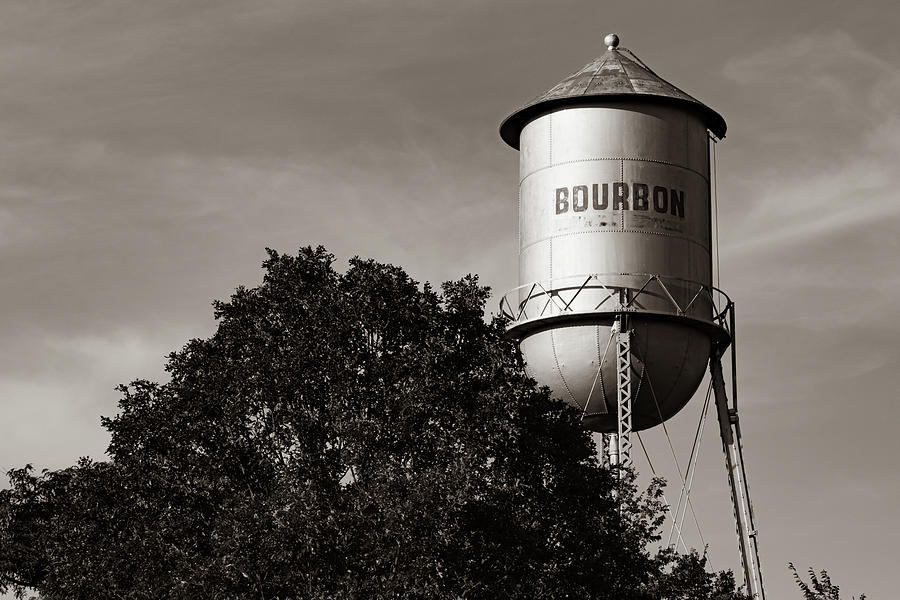This black and white photograph captures a prominently positioned metal water tower labeled "BOURBON" in capital black letters. The water tower, supported by four metal poles, features a distinctive triangular roof with a ball at its peak. The background showcases a dark, cloudy sky, indicative of an impending storm. To the left of the water tower, a large, leafy tree partially obscures the base of the structure. The tree's foliage, though indistinguishable in color due to the black and white format, appears dark and substantial, almost fluffy. There are no other elements, such as people or animals, in the image. The overall scene conveys a stark and somewhat somber atmosphere with the interplay of the looming water tower, the substantial tree, and the ominous cloudy sky.